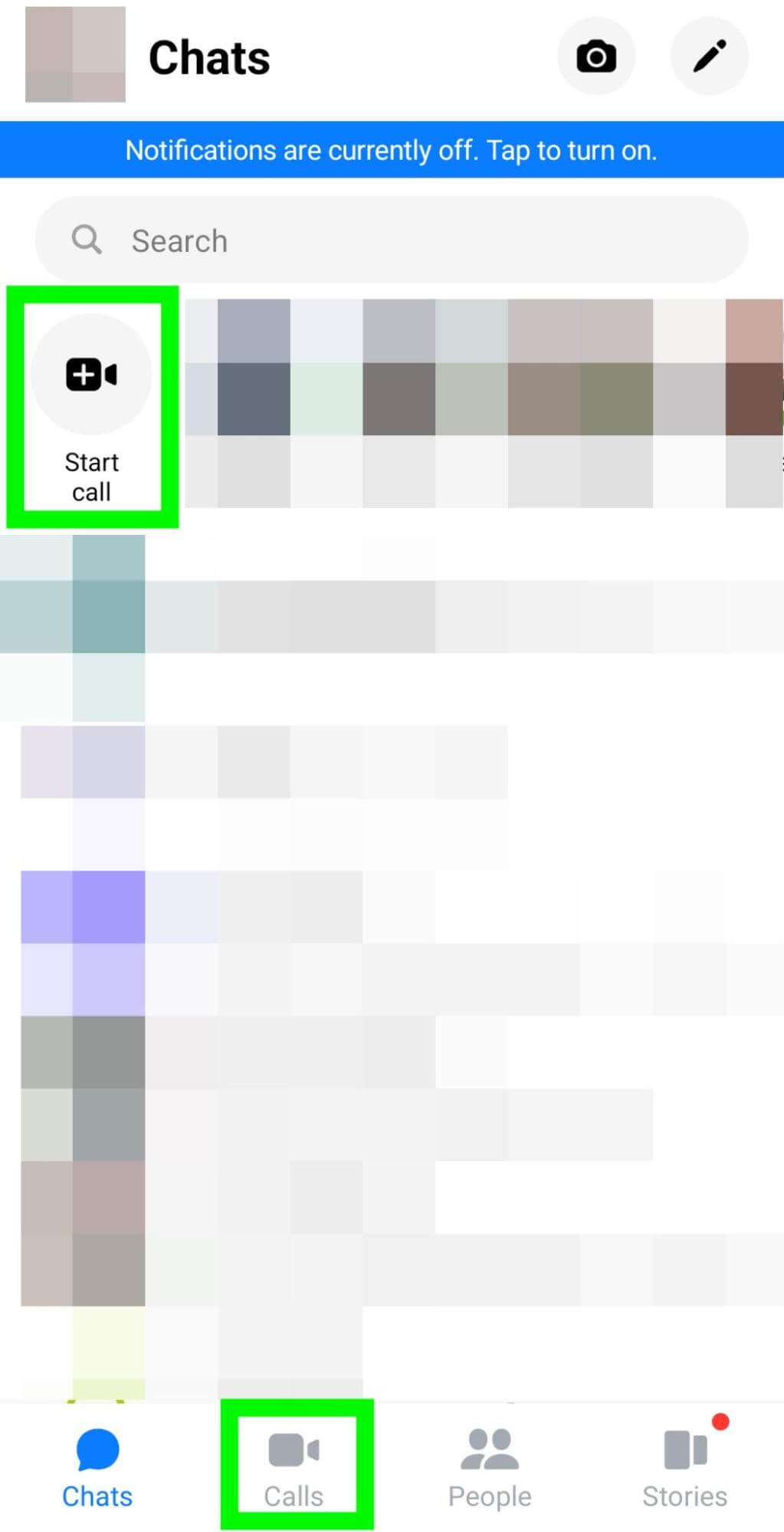The image appears to be a screenshot of a messaging app interface, possibly WhatsApp or a similar application. The interface is organized as follows:

- **Top Section**:
  - In the upper left corner, there's an icon consisting of smaller gray boxes in varying shades, likely representing pixel-like elements. Beside this icon, the word "Chats" is displayed in black text.
  - In the upper right corner, there are two icons within circles with gray backgrounds. The first icon is of a black camera, indicating a camera or photo function. The second icon is of a black pen or pencil, suggesting a writing or editing function.

- **Middle Section**:
  - Below these icons, there's a prominent blue rectangle centered in the screen. The rectangle contains white text stating, "Notifications are currently off. Tap to turn on."
  - Directly beneath the notification rectangle is a search bar with a magnifying glass icon and the placeholder text "Search."
  
- **Main Content Area**:
  - On the left side of this section, there's a green-bordered rectangle with a circular gray icon inside it. The icon depicts a video camera, and below it, the text "Start Call" is displayed.
  - Next to the "Start Call" button, there are various squares in a mix of colors, predominantly shades of gray with a few red-tinted squares. This pattern continues down the screen with additional squares in shades of blue, gray, and white.

- **Bottom Navigation Bar**:
  - At the bottom of the page, there are labels and icons for different sections of the app: "Chats," "Calls," "People," and "Stories." The "Calls" section is highlighted with a green border. Additionally, the "Stories" section has a red dot above it, possibly indicating new activity or updates.

The layout and elements suggest an interface for managing conversations, calls, and social stories within a messaging application.